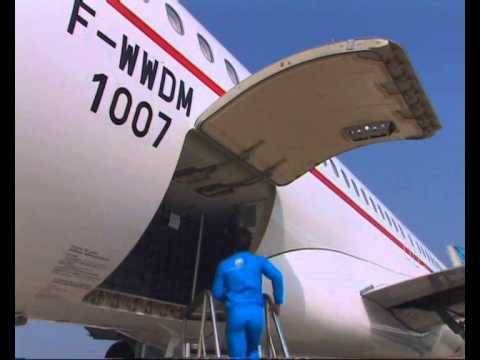The photo captures a scene set outdoors against a clear, medium-blue sky, featuring a close-up of a white commercial airplane with a red stripe along its side. Black text reading "F-WWDM 1007" is prominently displayed beneath the stripe. In the foreground, a plane technician, dressed in a medium-blue uniform, stands on a stepladder, facing away from the camera. He is inspecting the open undercarriage compartment of the airplane. The right wing and its wheel are partially visible at the bottom of the image. The technician's careful inspection suggests routine maintenance or safety checks are being conducted.